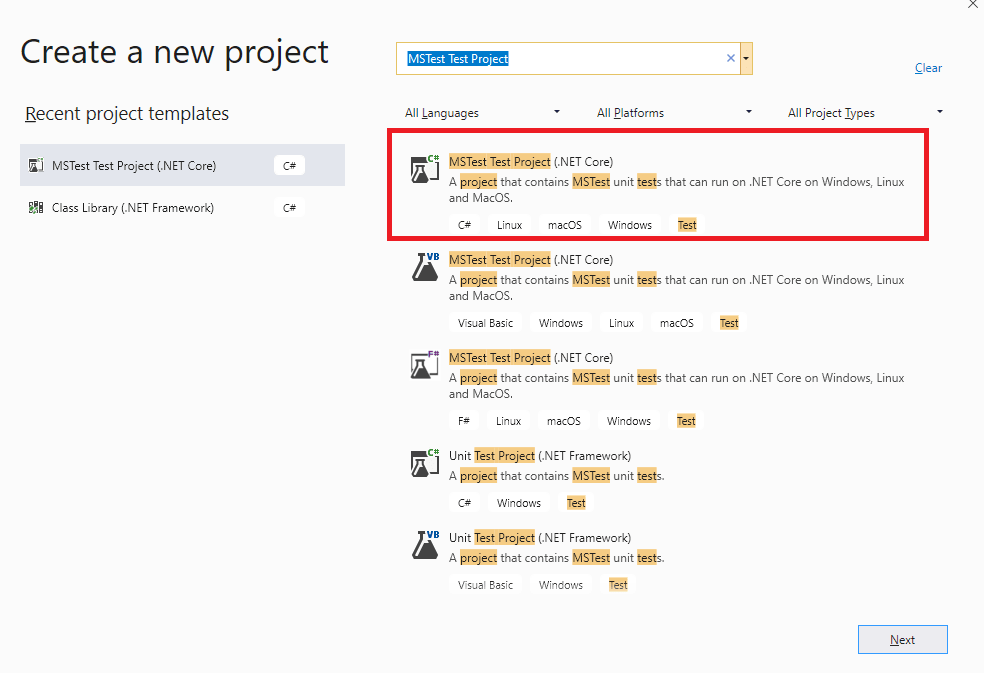The image features a user interface with a light gray background. In the upper left corner, there is text that reads "Create a new project." Below this heading, the text lists "Recent project templates," followed by "mstesttestproject.netcore" and "classlibrary.netframework." In the upper right corner of the image, there is an 'X' icon, typically used to close the interface.

Below the 'X' icon is a text box containing the text "mstesttestproject," which is highlighted in blue. Underneath this text box, there are filter options labeled "All languages," "All platforms," and "All project types."

Centered in the image is a rectangle with a red border. Within this rectangle, there is an icon resembling a beaker next to the label "mstesttestproject.netcore." A description follows, explaining that this is "A project that contains MSTest unit tests that can run on .NET Core on Windows, Linux, and macOS." Below this description, the tags "#Linux #macOS #Windows #Test" are displayed.

Further down, another beaker icon appears next to the label "mstesttestproject.netcore," followed by a similar description stating that this project also supports MSTest unit tests for .NET Core on multiple operating systems: Windows, Linux, and macOS. The description is followed by the tags "Visual Basic," "Windows," "Linux," "macOS," and "Test."

Subsequently, the text "mstesttestproject.netcore" is repeated once more. Below this repetition, the label "unittestproject.netframework" appears twice consecutively.

In the bottom right corner of the image, there is a button labeled "Next," indicating a step forward in the project creation process.